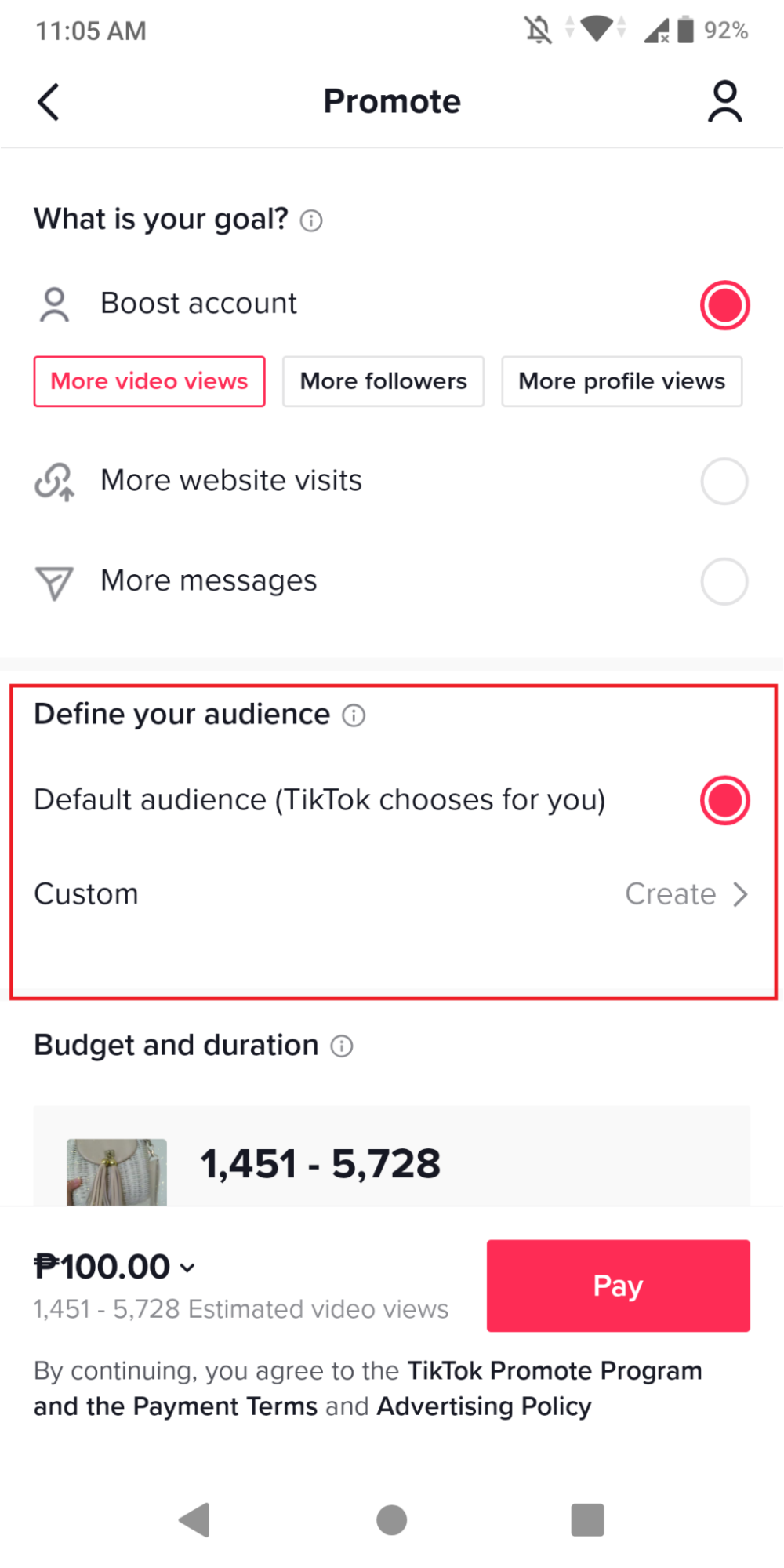Here’s a detailed and cleaned-up caption for the described image:

---

The image is a screenshot from a mobile phone, displaying a TikTok promotional settings interface. At the top left corner, the time is shown as 11:05 AM, with additional symbols to the right indicating various phone statuses, including a disabled alarm, full signal strength, and a battery life of 92%. Below the status bar, the navigation header features a back arrow on the left, the word "Promote" in the center, and a profile icon on the right.

Directly beneath the header, the interface prompts the user with the question, "What is your goal?" accompanied by an information icon. Below, there is a section highlighted with a red circle around a profile icon labeled "Boost Account." Within this section are three selectable options for promotional goals: 
1. "More video views" (highlighted in red)
2. "More followers"
3. "More profile visits"

Under these options are two additional, unchecked options:
1. "More website visits"
2. "More messages"

Further down, a red-highlighted box labeled "Define your audience" is visible, including a selected radio button for "Default Audience - TikTok chooses for you." There is also an option for customizing the audience with a link to "Create."

Below this section, outside the red-highlighted box, the interface features "Budget and Duration" settings. An estimated range "1,451 to 5,728" is displayed, likely indicating an estimated budget or currency range. Below this, it says "1,451 to 5,728 estimated video views." A red "Pay" button is positioned adjacent to this range.

---

This caption encapsulates the detailed elements in the described screenshot, providing a comprehensive understanding of the interface and its options.